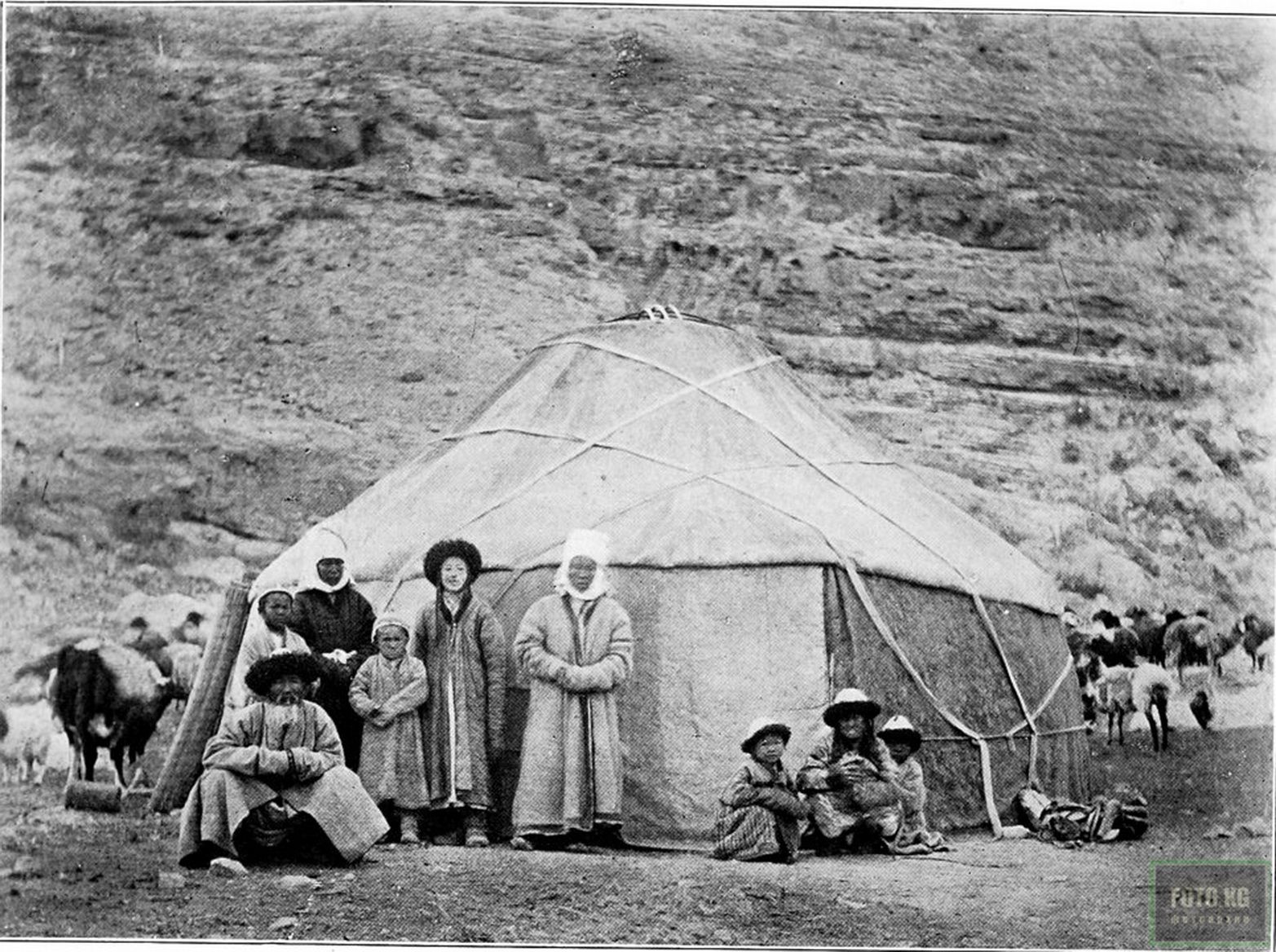This black and white, grainy photograph features a large, tent-like structure set up in a dry, rocky area close to a mountain. The tent, which almost reaches the size of a small house, appears to be cone-shaped and possibly covered in burlap. In front of the tent stands a group of nine individuals, comprising five adults—including one senior, an elderly man with a beard wearing a circular hat—and four children. All figures are dressed in distinctive, non-Western overcoats and jackets, with atypical hats. The scene also includes visible livestock, such as cattle and sheep, positioned both beside the tent and in the background. The bottom right corner of the image has a watermark with the initials "FKG" in white text inside a black box with a green outline. The overall setting suggests a native tribe, possibly Mongolian, against the backdrop of a towering stone cliff and a dirt-covered ground.